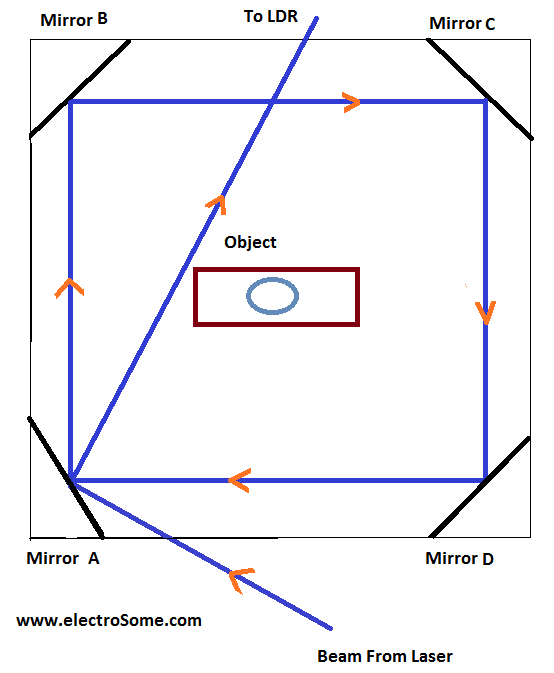The image is a detailed diagram of a laser beam pathway within a square arrangement of mirrors, all depicted on a white background. At the bottom left corner, there's a label with the website, "www.electrosome.com." The laser beam initiates from the bottom of the image, marked by the text "Beam from Laser," and is shown with a blue line extending upwards to Mirror A, located in the lower left corner. The beam then reflects at a 90-degree angle and travels across the square room, sequentially bouncing off mirrors positioned in each corner. 

In the upper left corner, Mirror B is indicated with black labeling, similarly, in the upper right corner is Mirror C, and Mirror D is positioned at the bottom right corner. These mirrors guide the beam in a square path, finally directing it towards the center, labeled "2LDR." Additionally, within this central square, there is a red rectangle that encloses a pale gray oval, with the word "Object" placed above it in black text.

Blue lines, representative of the beam, trace a path that intersects each mirror in the specific sequence (A, B, C, D) and continue further in diagonal patterns. These lines creatively form small triangles at each corner of the black square outline and create intersecting paths within the central diagram. Adjacent to these paths, various geometric symbols like greater than and less than signs can be observed.

Overall, this intricate schematic showcases the journey of a laser beam through a mirrored setup, ultimately highlighting the reflection sequences and object placement within a confined space.